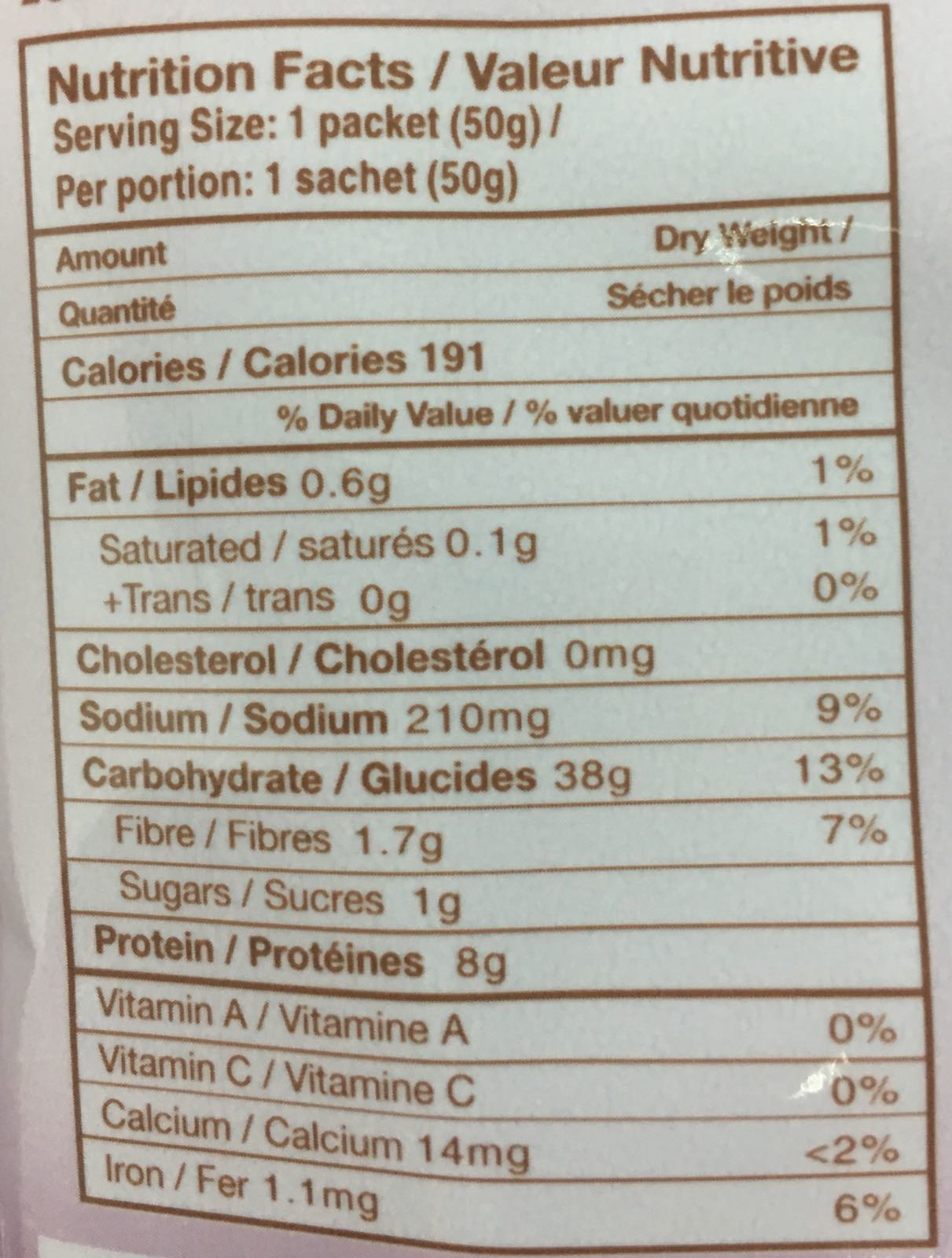This detailed image captures the nutrition facts label found on the back of a package. The label is predominantly white with text displayed in both English and French, separated by slashes. Encased in a brown-bordered box, the label's content is divided by brown horizontal lines for clarity. At the top, it reads "Nutrition Facts / Value Nutritive." Below that, the serving size is specified as one packet (50 grams) / "Portion: 1 sachet (50 grams)."

The nutritional breakdown is presented as follows:

- Calories: 191
- Fat / Lipides: 0.6 grams
- Cholesterol: 0 mg
- Sodium: 210 mg
- Carbohydrate: 38 grams
- Protein: 8 grams

Additionally, the label provides information about the quantities of certain vitamins and minerals:

- Vitamin A: 0%
- Vitamin C: 0%
- Calcium: Less than 2%
- Iron: 6%

The specific French translations are consistently provided alongside the English terms, ensuring clear and comprehensible information for bilingual consumers.